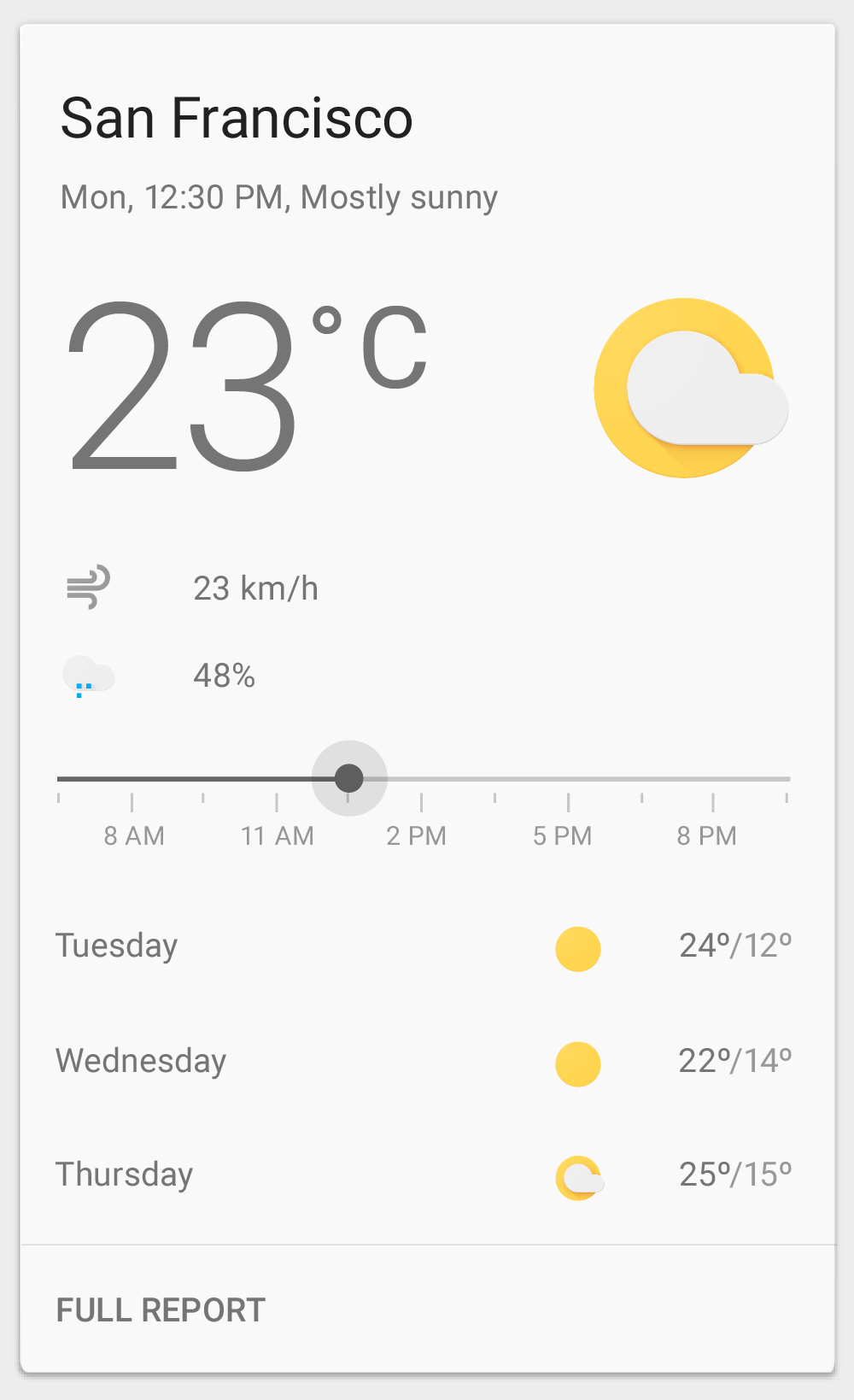Screenshot of a weather app for San Francisco at 12:30 p.m. on a Monday. The interface has a vertical rectangular shape typical of a smartphone screen, with a white background and primarily black text. At the very top, it displays "San Francisco" followed by "Monday, 12:30 p.m." The forecast for the current moment is "Mostly Sunny" with a temperature of 23°C. To the right of the temperature is an icon of a yellow sun containing a white shape, possibly indicating some cloud cover.

Beneath the temperature, there's a symbol indicating wind speed, showing "23 km/h." Further down, a symbol representing rainfall shows three small blue squares with "48%" next to it, indicating precipitation chances. Below this section, there's a timeline displaying weather predictions at intervals from 8 a.m. to 11 a.m., 2 p.m., 5 p.m., and 8 p.m.

Following the timeline, there's a forecast for the upcoming days. Tuesday shows a sun icon with temperatures of "24°C / 12°C." Wednesday also has a sun icon, indicating "22°C / 14°C." Thursday features a partially covered sun icon with temperatures listed as "25°C / 15°C." At the very bottom, the option "Full Report" invites users to access more detailed weather information.